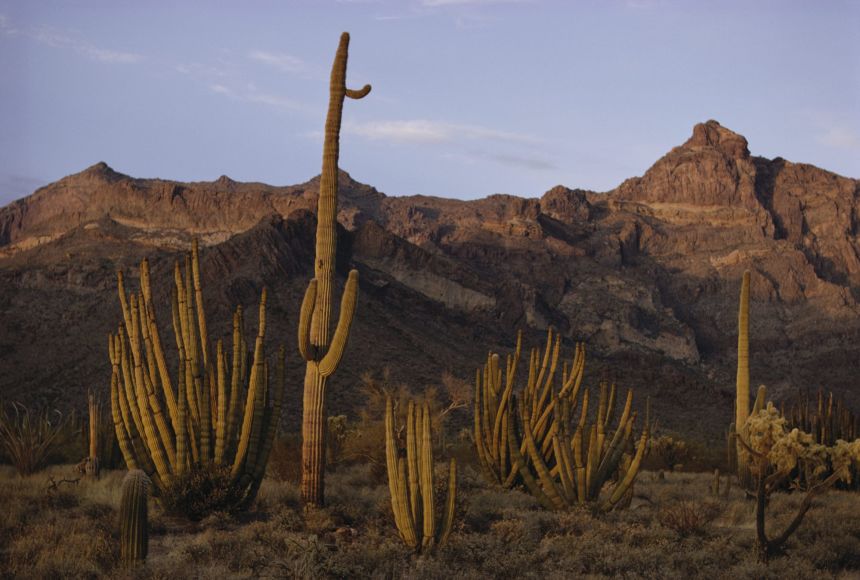This detailed photograph captures a quintessential desert scene in the United States during the evening around sunset. The focal point features several distinct types of cacti, predominantly including a couple of tall, thin saguaro cacti and three or four organ pipe cacti with numerous thin, arm-like extensions. There is also a notable presence of a teddy bear cholla cactus in the bottom right. The ground is dry and sprinkled with sparse, dead-looking desert foliage and grasses, accentuating the arid environment. In the background, rugged, rocky mountains exhibit varying shades of brown and tan, with the top third bathed in the warm glow of the setting sun while the lower portions linger in shadow. The sky overhead shifts between pale blue and purplish hues, dotted with thin, wispy stratus clouds, contributing to the tranquil ambiance of this cooling desert evening.